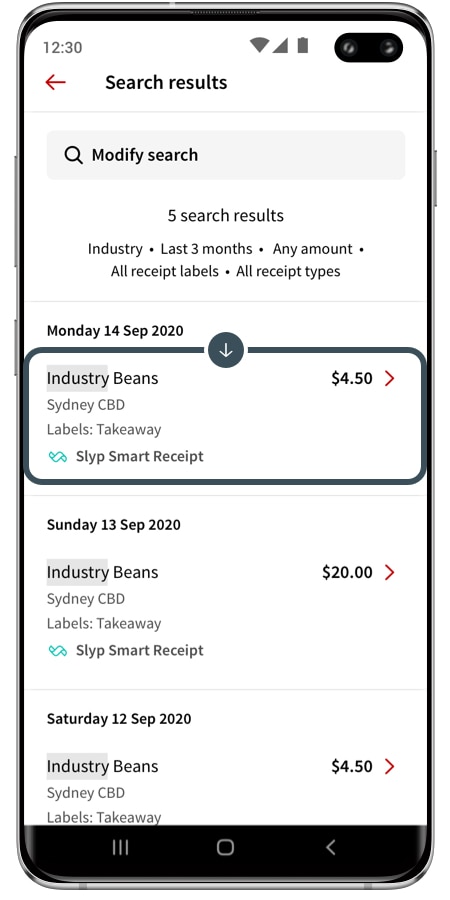**Detailed Caption:**

The screenshot displays a search results page with a total of 1,230 entries indicated by a red arrow pointing to the left. At the top, there is a search bar accompanied by a magnifying glass icon, labeled "Modify Search." The search has been refined to show results based on the following criteria: industry within the last three months, any amount, all receipt labels, and all receipt types.

The results are as follows:

1. **Monday, 14th September 2020:**
   - Search narrowing options involve "Industry: Beans"
   - Specific criteria highlighted: "Sydney CBD" in all capital letters
   - Labels: "Takeaway"
   - Receipt Type: "Slip Smart Receipt (SLYP)"
   - Total Amount: $4.50

2. **Sunday, 13th September 2020:**
   - Search narrowing options involve "Industry: Beans"
   - Specific criteria highlighted: "Sydney CBD" in all capital letters
   - Labels: "Takeaway"
   - Receipt Type: "Slip Smart Receipt (SLYP)"
   - Total Amount: $20.00

3. **Saturday, 12th September 2020:**
   - Search narrowing options involve "Industry: Beans"
   - Specific criteria highlighted: "Sydney CBD" in all capital letters
   - Labels: "Takeaway"